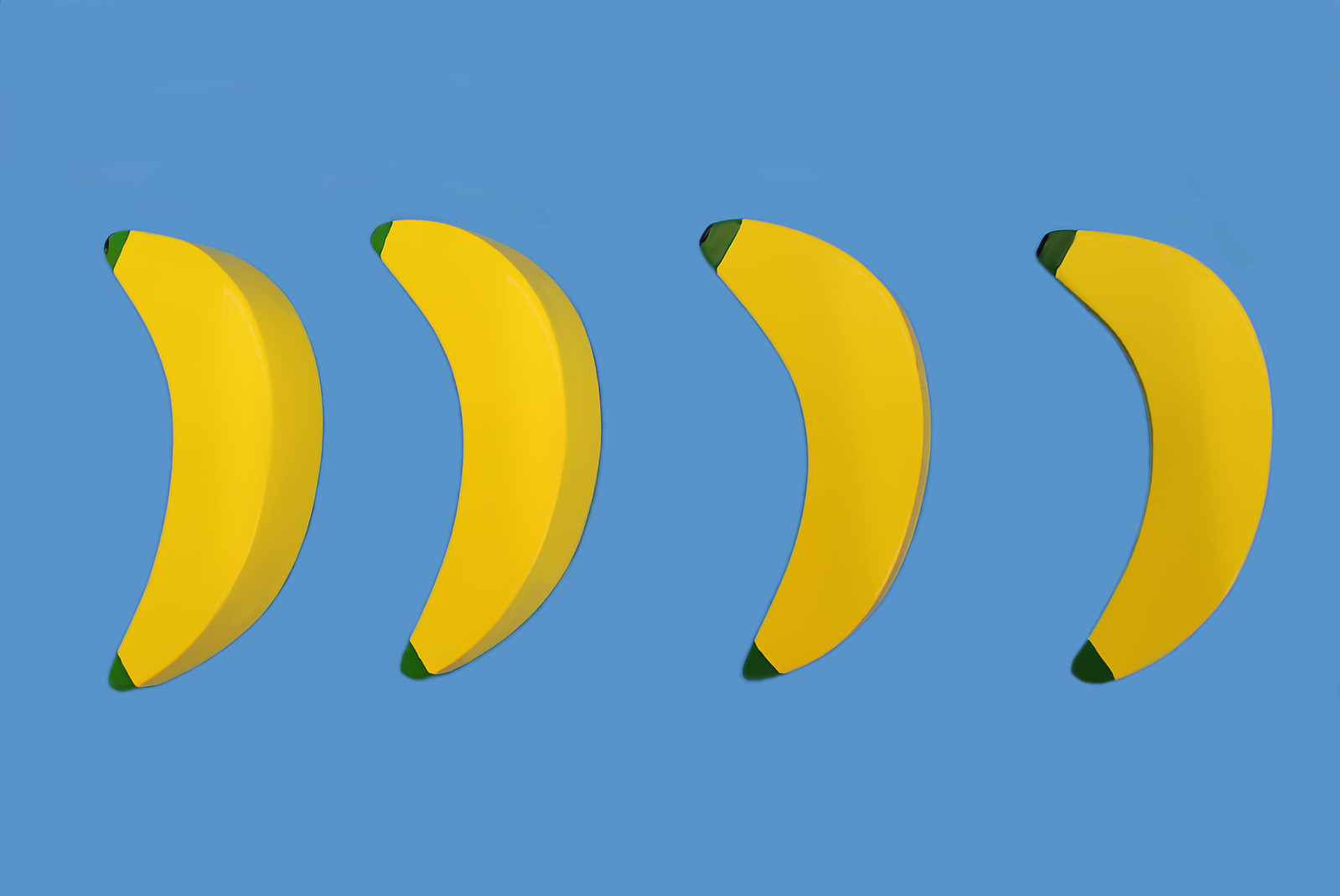This landscape-oriented, computer-generated illustration features a vivid arrangement of four bright yellow bananas set against a baby blue background. The bananas are aligned side by side, all elegantly curved to the left. Notably, the first two bananas on the left are nearly identical with matching lengths of green caps at both ends. The latter two bananas share a similar appearance but with thicker, darker green caps. Each banana has distinct dark brown tips, varying slightly in size. The bananas exhibit a subtle depth, hinted at by thin, shadowed edges along their curves, enhancing the visual composition. The overall simple yet striking design creates a pleasing contrast against the background, with no accompanying text or descriptions to detract from the visual focus.